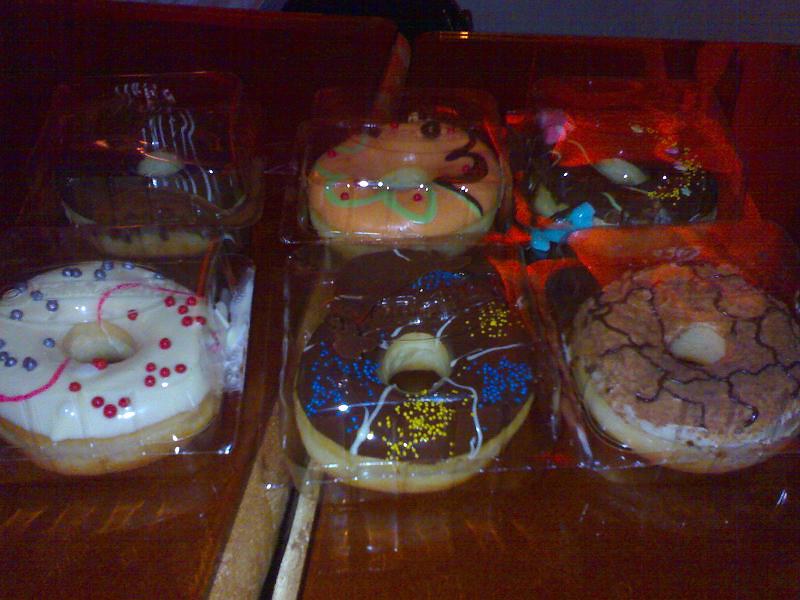This color photograph showcases six individually wrapped, elaborately decorated doughnuts, arranged in two rows of three on a dark wooden surface. The wooden surface seems to have a lighter, off-white trim, contributing to the detail in the photo. The doughnuts are inside a bakery display case or under some plastic covering, where reflections make it a challenge to discern all the intricate decorations clearly.

Starting from the back row, the leftmost doughnut is not fully visible but potentially features purple and white striped frosting, possibly resembling a blueberry muffin. The middle back doughnut is adorned with vibrant orange frosting, a pale green flower around the doughnut hole, red dots, and a swirl of chocolate. The rightmost doughnut in the back row is mostly obscured but appears to have a chocolate base.

In the front row, from left to right: the leftmost doughnut is white frosted with red and blue candy dots and a pink swirl. The center front doughnut has chocolate frosting, decorated with blue and yellow sprinkles, and several white streaks. The front right doughnut has a tan or latte-colored frosting with crumb-like texture and purple lattice-like squiggles.

Despite the dim lighting and reflections, the assorted colors and designs of the doughnuts add an artistic and appetizing appeal.